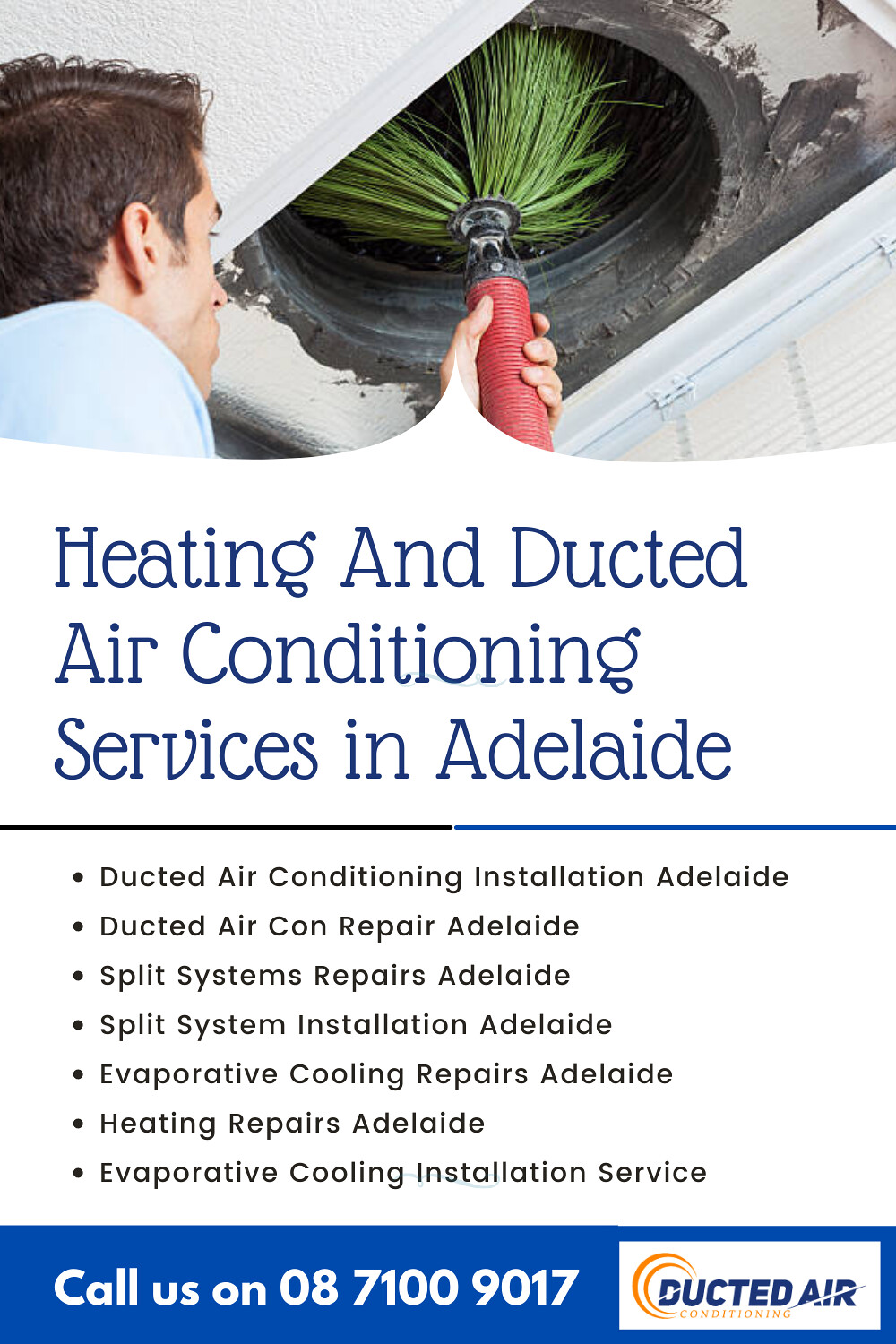The advertisement is for a heating and air conditioning service in Adelaide. The top portion features an image of a professional-looking man with brown hair, cleaning an air duct using a red-handled apparatus equipped with green bristles. The background of the image shows the duct opening, emphasizing the cleaning process. Below the image, large blue text on a white background declares "Heating and Ducted Air Conditioning Services in Adelaide." Beneath this heading, a list of services is presented, highlighting: Ducted Air Conditioning Installation Adelaide, Ducted Air Conditioning Repair Adelaide, Split Systems Repair Adelaide, Split System Installation Adelaide, Evaporative Cooling Repairs Adelaide, Heating Repairs Adelaide, Evaporative Cooling Installation Service. At the bottom of the ad, a blue banner with white lettering provides contact information, saying, "Call us on 08-7100-9017." Additionally, the company's logo, reading "Ducted Air Conditioning," is prominently displayed.